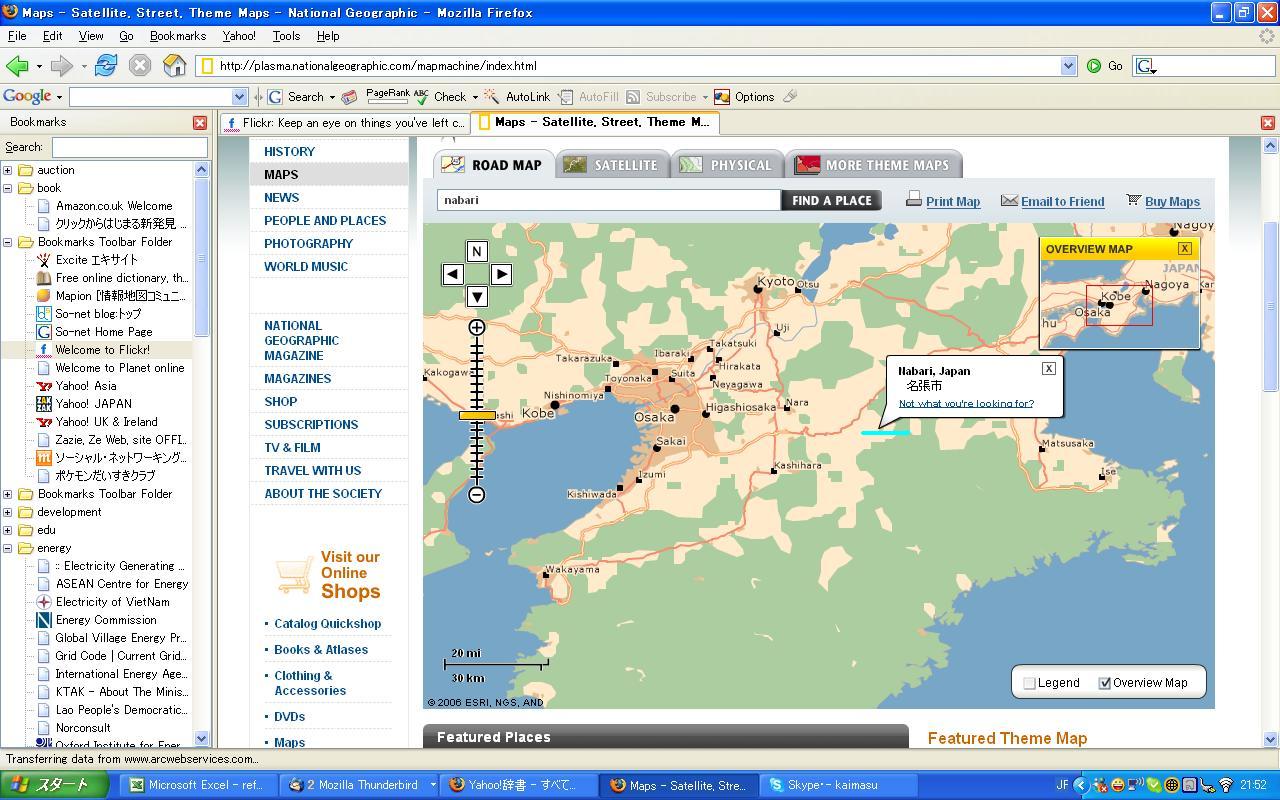The photograph is a color screenshot of a computer screen displaying a web browser that resembles Microsoft Edge. Dominating approximately 80% of the image on the right side is a detailed map, which appears to be of a location in Japan. The map exhibits a legend and features Japanese characters, providing additional context and information. Various map settings and themes such as "National Geographic" are available in a sidebar on the left. Above the map, there are tabs that allow the user to switch between different views including satellite and physical modes. An overlay in the upper right corner of the map provides a compact overview. To the far left, there is a column reminiscent of an email list, which includes both English and Japanese text. This column seems designed for organizing various information. Above the entire interface, a prominent bright blue banner runs across the top, indicating the active browser window for the map application.